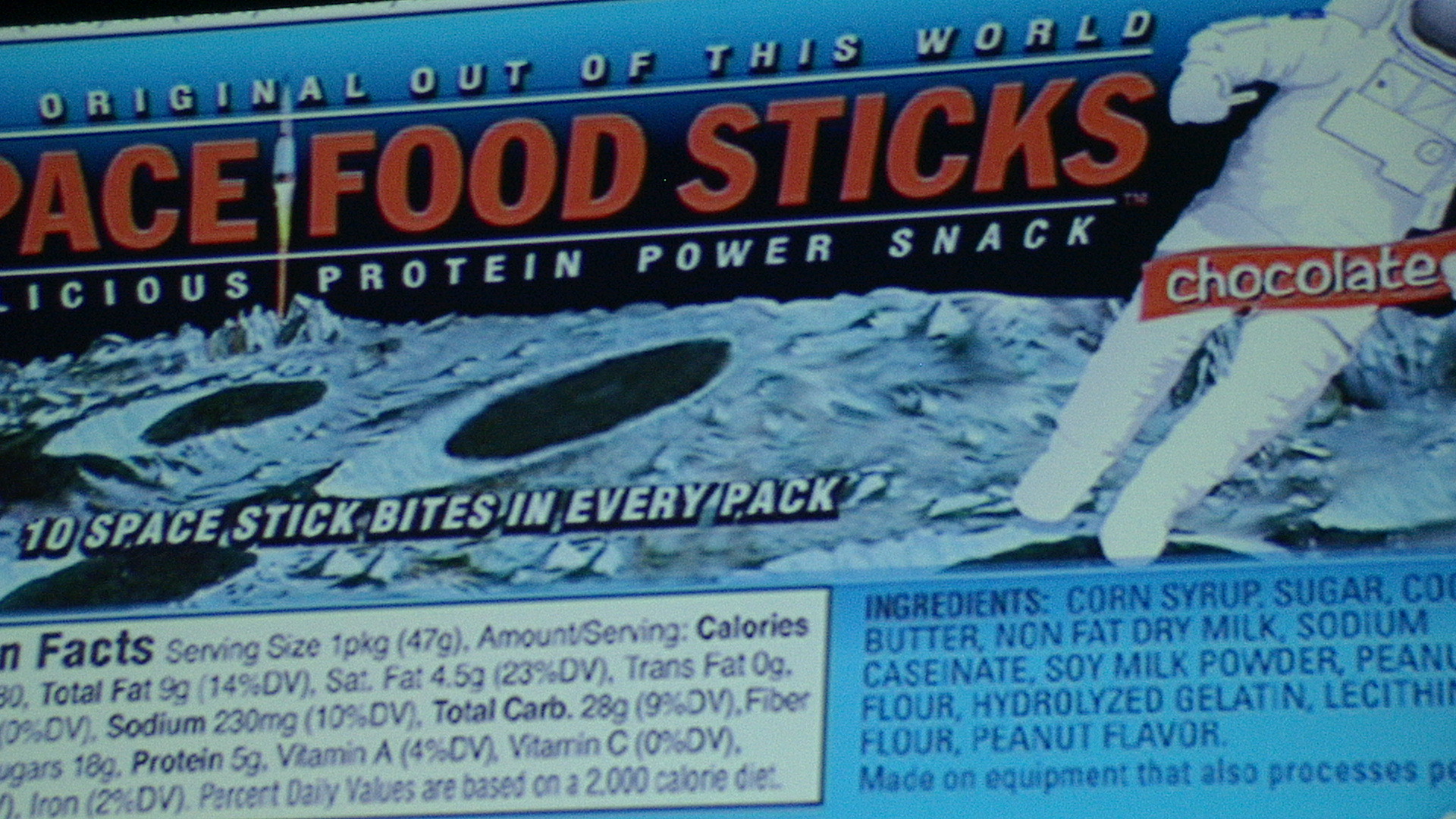This photograph captures a vintage-style food package for "Space Food Sticks." The packaging is a visually appealing blue cardboard box adorned with a detailed close-up image of the moon, showcasing its craters and surface texture. Enhancing the nostalgic space theme, a cartoon astronaut in a classic white uniform and helmet can be seen walking on the moon's surface. The front of the box proudly displays the tagline, "The Original Out-of-This-World Delicious Protein Power Snack," emphasizing its unique appeal. A vibrant red banner declares the flavor as chocolate, further enticing potential consumers. The package also informs buyers that each pack contains 10 space stick bites. Included on the box are sections detailing the nutritional facts and a list of ingredients, which include corn syrup, sugar, butter, and nonfat dry milk, providing a comprehensive overview of the product.